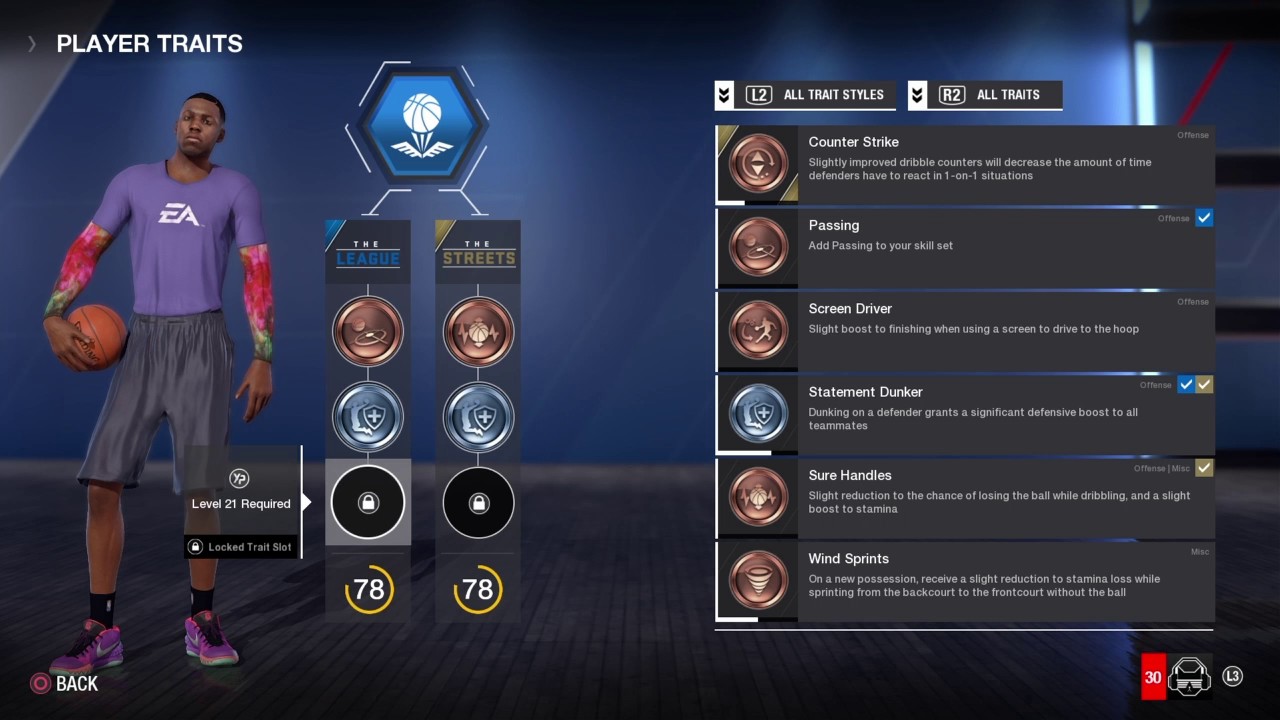A detailed screenshot of a basketball game’s player traits selection page. At the top left, the header "Player Traits" sits above an image of a young African American man holding a basketball in his right hand. He is dressed in a bluish-purple shirt with the letters "EA" emblazoned on it, paired with dark-colored shorts and athletic shoes that are predominantly purple with other mixed colors.

To the right of this image, there's an icon of a basketball followed by two columns: "The League" and "The Streets." Each column contains images in three rows. The top row features a circle with a copper-colored background. The second row contains a silver background with an image of a basketball player inside it. The final row displays a circle with a black background and an icon of a padlock, under which it states "Level 21 Required - Locked Trait Slot" and the number 78 is listed as the final entry in both columns.

On the right side of the page, the headings "All Trait Styles" and "All Traits" are visible. Under these headings, various categories are listed including Counter Strike, Passing, Screen Driver, Statement Dunker, Sure Handles, and Win Sprints. Each category comes with a brief description of its function. For instance, "Passing" is described as "Add passing to your skill set," while "Screen Driver" notes "Slight boost to finishing when using a screen to drive to the hoop."